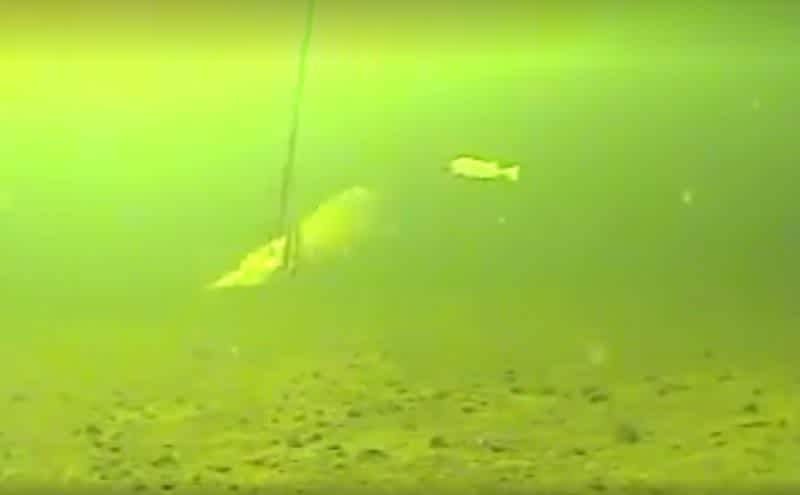The rectangular underwater photograph showcases a murky and polluted body of water, with a predominant palette of tan green, lime green, and hints of yellow. The scene is hazy, making it difficult to discern the precise nature of the environment, whether it is a lake or an ocean. The sandy bottom is sprinkled with pebbles and rocks, giving the impression of a shallow area. From the top of the frame, a rope or fishing line descends, with an ambiguous white object, akin to a piece of bait, tied to it. Nearby, the indistinct silhouette of a small fish is visible, further emphasizing the cloudiness of the water. The overall impression is one of murkiness, pollution, and underwater obscurity.